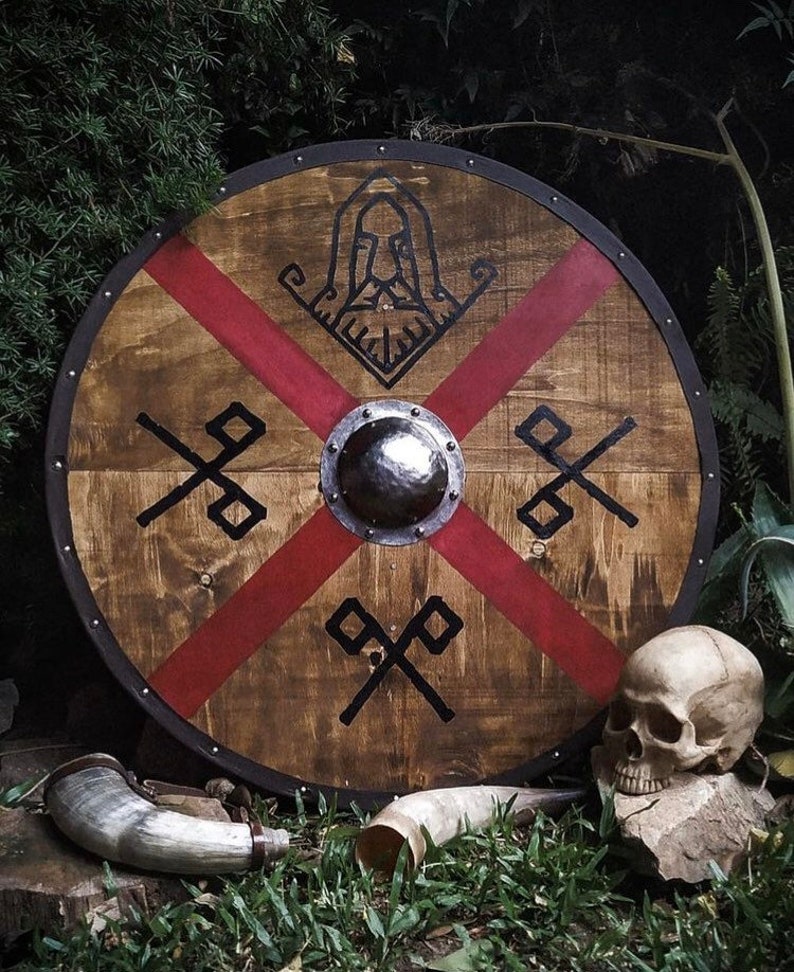In a dimly lit forest setting, a Viking shield stands prominently propped against dense shrubbery. The shield, centered in the image, is crafted from wood and encircled by a black metal band affixed with nailheads. Divided into four quadrants by a bold red X, the shield's central feature is a silver dome. The top quadrant showcases a lined illustration of an older man with a mustache and hood, rendered in black. Each of the three lower quadrants contains a similar design, resembling crossed flags or horns. In the foreground, among the sparse grass, lie two horns and a rock topped with a human skull facing the image center, adding to the scene's haunting medieval ambiance.